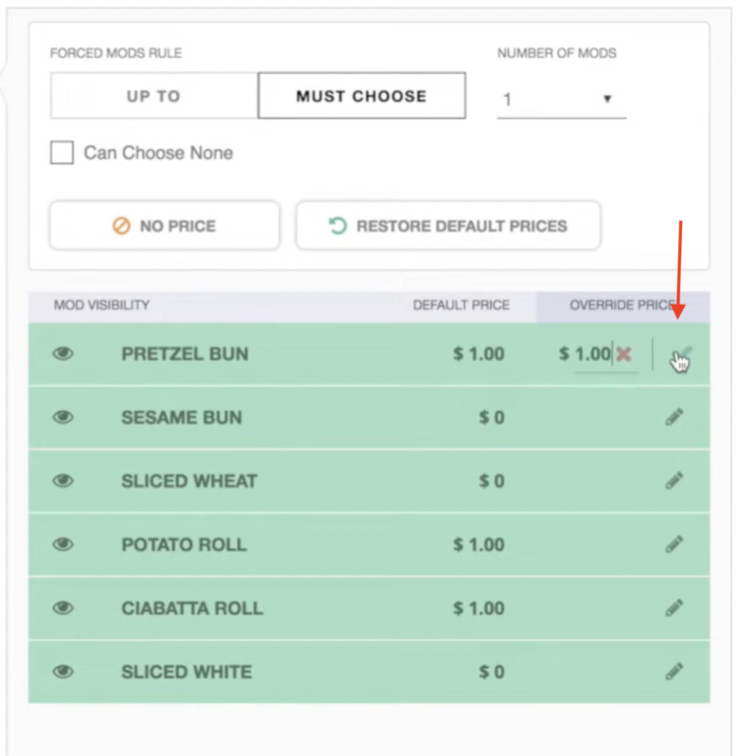The image displays a webpage featuring a detailed form interface for selecting bread options with customizable rules. The top of the form includes the heading "First Mods Rule," and below it, the text "Must Choose" is highlighted, indicating that it has been selected as the sorting rule. Additionally, the "Number of Mods: One" option is visible, and the checkbox for "Can Choose None" is unchecked, implying that at least one selection must be made. 

The visible options for bread include the following, each paired with its respective price:
- Pretzel Bun: $1
- Sesame Bun: $0
- Sliced Wheat: $0
- Potato Roll: $1
- Ciabatta Roll: $1
- Sliced White: $1

There is a button that reads "Restore Default Prices," likely intended to reset any price adjustments made by the user. The interface uses a color scheme featuring white, grey, black, and green, all set against a primarily white background for clarity and readability.